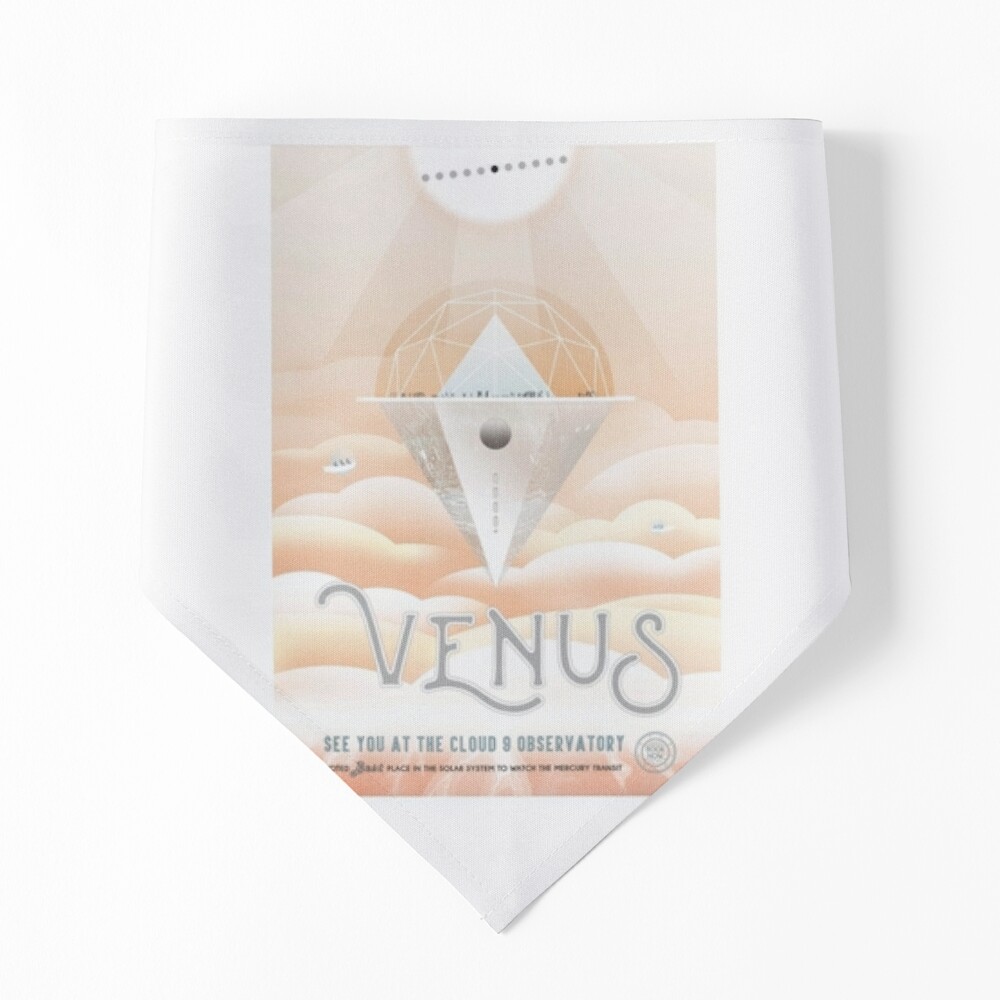The image features a large, off-white square background with no discernible borders, creating a seamless look. Placed at the center of this background is an object resembling a piece of fabric or a folded napkin, tapering downwards to a V shape, much like the tip of a tie or a handkerchief emerging from a pocket. This object is white and displays subtle stitching along its edges. 

In the middle of this object, there is a vertical rectangular panel showcasing an artistic design. The design features a conical-shaped floating platform with a semi-spherical glass dome on top, positioned above a picturesque scene of billowy, peach-colored clouds reminiscent of those seen from above. The dome and platform are accentuated with intricate white lines forming geometric patterns. Below this imagery, there is text written in elegant, curvy, silver-gray letters that reads "Venus." Further down, in the same stylish font, the caption says, "See you at the Cloud 9 Observatory." The entire arrangement is aesthetically pleasing, casting a delicate shadow on the serene background.